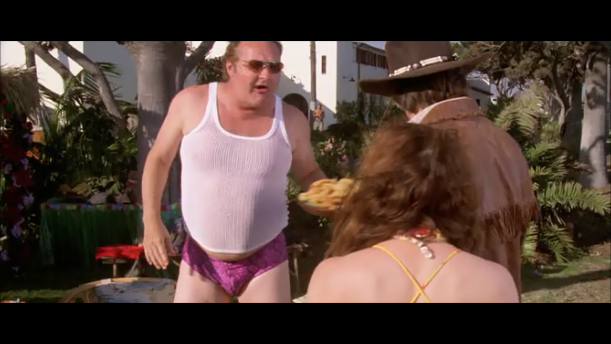The image is a scene from a movie depicting three individuals in an outdoor setting, possibly someone's tropical yard. In the foreground, a man who resembles Randy Quaid is dressed in a white tank top and pink-purple bikini underwear, revealing his bare legs. He wears sunglasses and holds an object in his left hand. To his right, a woman with flowing, curly red or brown hair, has her back to the camera. She wears a top with thin yellow spaghetti straps, suggesting a bikini. Positioned above her to the right is a man sporting a brown cowboy hat with beads, short brown hair, a black leather coat with fringes, and a white band around the hat. They all appear to be conversing amidst a backdrop of lush vegetation, including palm trees, and a white building. The setting is vividly detailed with various colors such as pink, purple, brown, yellow, green, and white, enhancing the tropical, laid-back atmosphere.